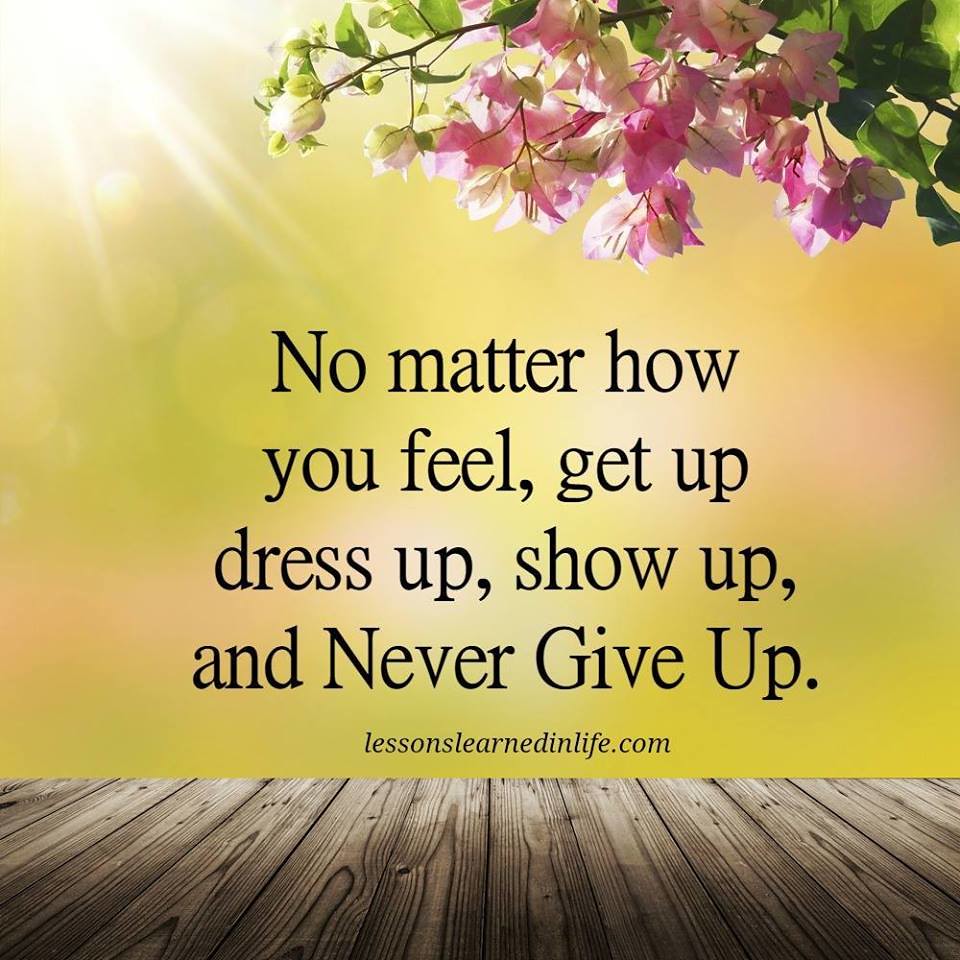The image is a large, square, colorful piece that conveys an inspirational message often seen on motivational posters or social media memes. The background features a bright golden sky, with the sun's rays shining through in the upper left-hand corner, casting a warm, radiant glow. Adorning the middle and upper right-hand corners are clusters of beautiful flowers in shades of white and pink, accompanied by lush green leaves; some flowers are in full bloom while others are still budding. Dominating the center of the image, printed in bold, black text, is the motivational quote: "No matter how you feel, get up, dress up, show up, and never give up," with the letters N, G, and U in "never give up" capitalized for emphasis. Below this quote, in smaller text, is the website attribution: "lessonslearnedinlife.com." Adding to the composition, the bottom section of the image features vertically aligned wooden boards, reminiscent of a boardwalk, with distinct wood grains and shades of brown. The overall background is a warm blend of bright yellow, interspersed with hues of pink and orange, creating a vibrant and uplifting visual.